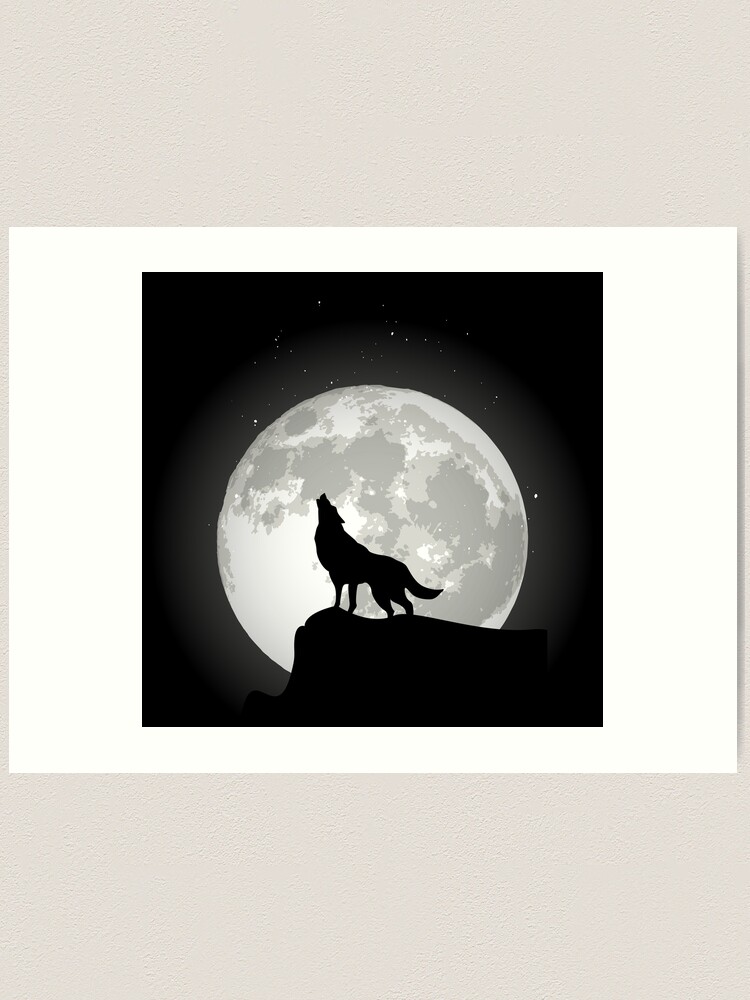The image depicts a Halloween-themed painting mounted on a white wall. The painting, enclosed in a bright white frame that contrasts with the wall's duller white, features a black square centered within it, symbolizing the night sky. Dominating the scene is a meticulously detailed, luminous white moon, occupying the middle section of the composition and revealing gray craters on its surface. Emanating light, the moon creates a stark backdrop for the silhouette of a howling wolf, positioned on a rugged slab of rock at the moon's base. The wolf's body, estimated to be about six feet in length, is facing left with its head tilted upwards, howling towards the top left corner of the picture. Above the moon, a scattering of stars accentuates the nocturnal setting, merging with the moon's glow to evoke an eerie, cinematic atmosphere.